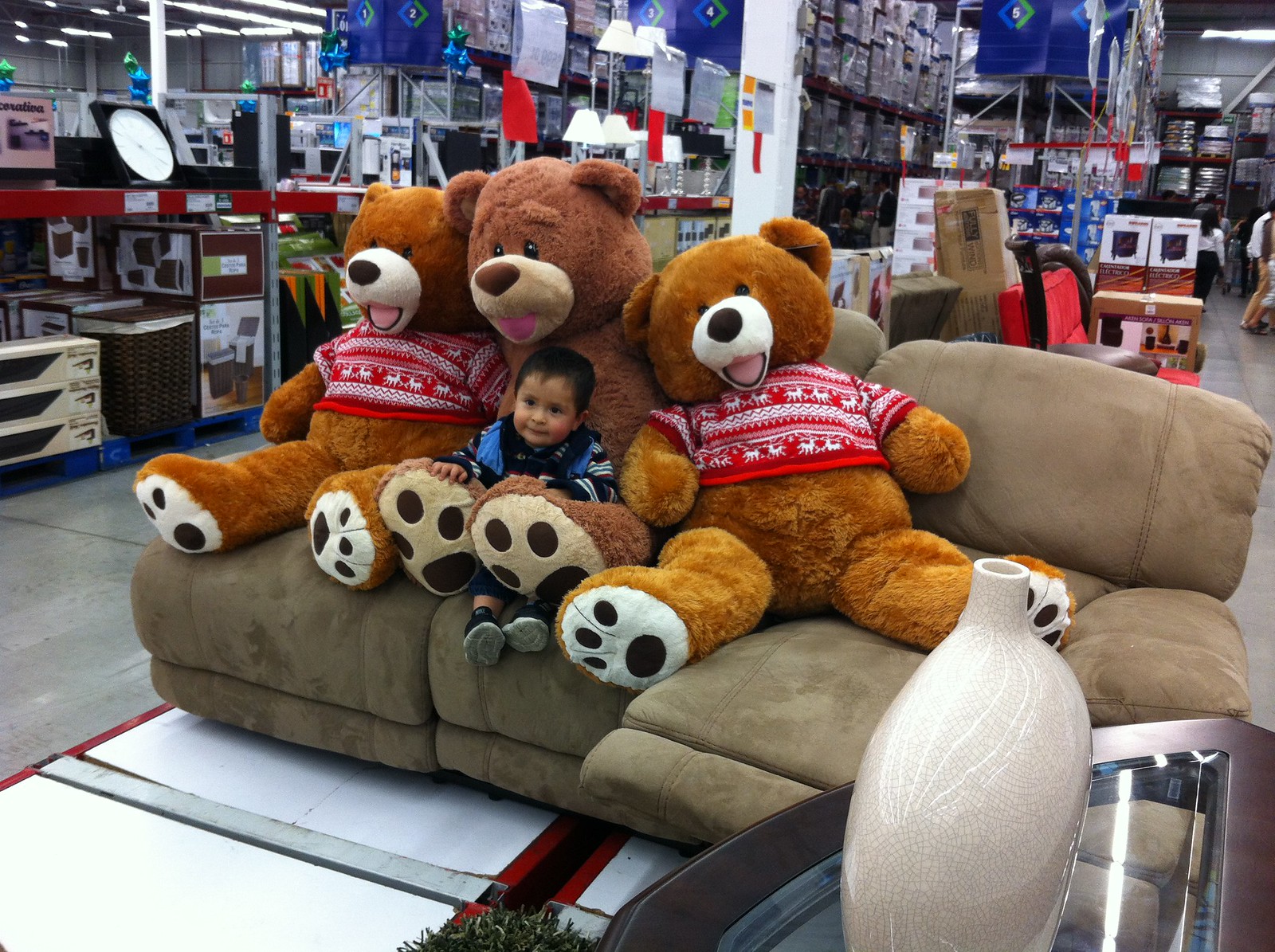In a bustling big box store, likely Sam's Club, the scene is set with six clearly marked aisles labeled one through six, grouped in pairs, each sign in distinctive blue with white numbering. The background is lined with display cases and merchandise, including shelves—with recognizable red accents—stacked with various unseen products. Featured prominently in the center of the image is a beige microfiber couch adorned with three enormous teddy bears, two auburn-colored ones flanking a darker brown bear. These teddy bears, each wearing cute red and white sweaters, dwarf a happy, young Hispanic boy with light brown skin and black hair, who is seated on the lap of the middle bear. The boy, dressed in a black and blue shirt, beams with joy, highlighting the playful interaction. On the lower right, a glass and silver coffee table holds a stylish white vase, grounding the cozy setup amidst the retail surroundings. To the left, an assortment of items including a clock are visible, adding to the everyday charm of this indoor store setting.